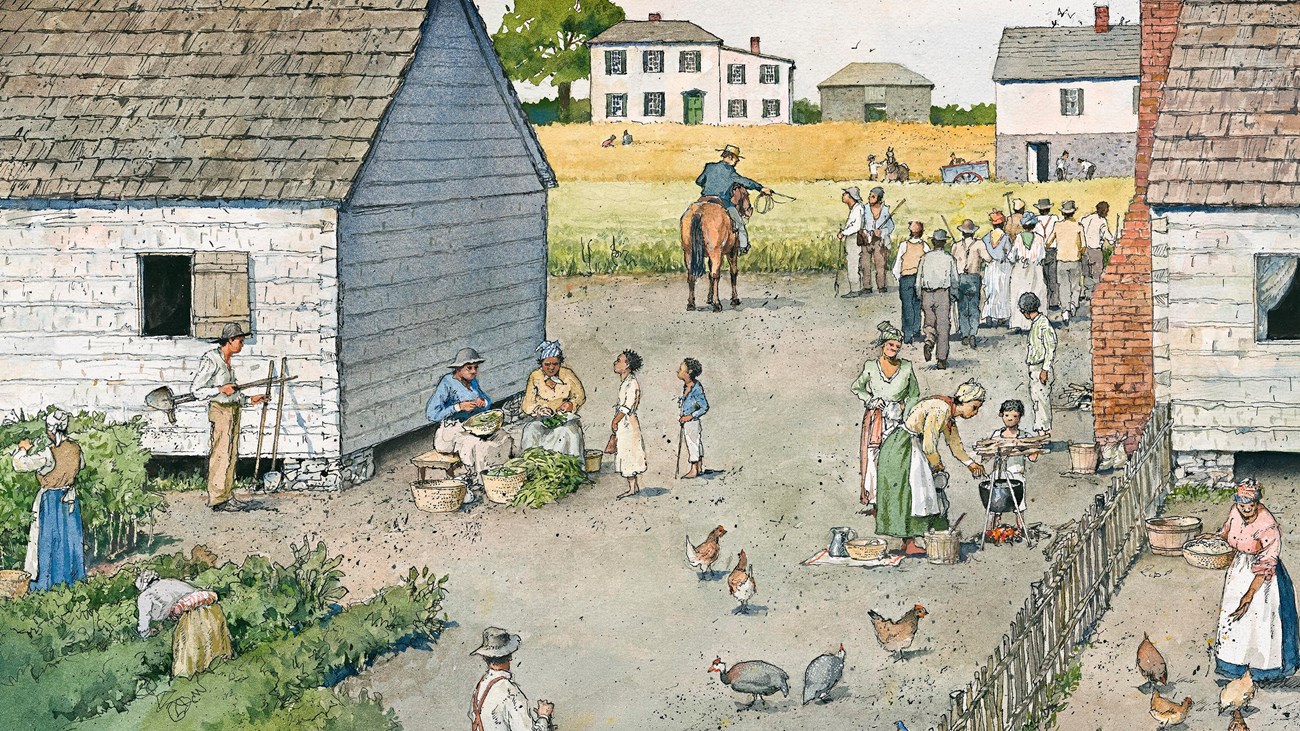The image is a detailed hand-drawn depiction of a bustling community, seemingly from many years ago, set in a farm-like village. Central to the scene is a man on horseback, wearing a distinctive blue suit jacket and a yellow top hat, pointing a stick at two people, likely indicative of his authority over them. The diverse activities suggest a community of workers, possibly slaves, engaged in various tasks. In the foreground, there is a gray courtyard where several groups are busy with different chores: a woman is picking bushes in the lower left corner, another trims bushes nearby, and two women assist a child over a cooking pot above a fire. Scattered throughout are people cooking with small fires, working in a vegetable garden, and feeding chickens. In the background, a large white house with a brown roof stands alongside a gray barn, beneath a gray sky with birds flying. A golden field stretches behind the barn, with two figures working the land near a person with a horse and wagon.